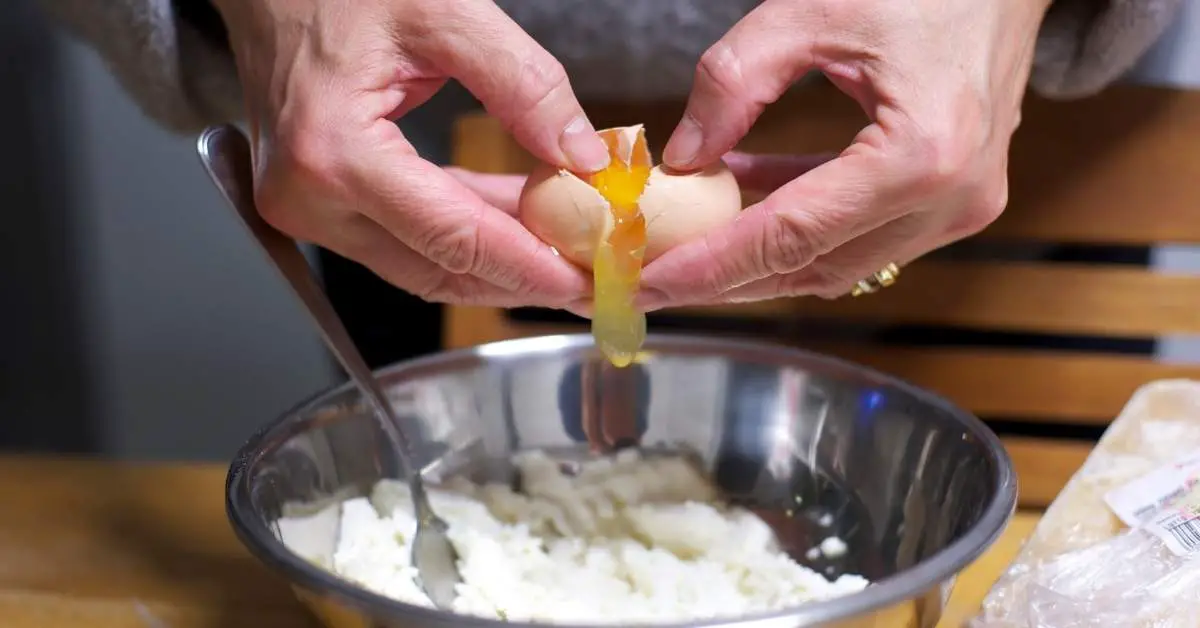In this detailed close-up image, a person is in the midst of cracking open a brown egg over a metal pan. Both of the person's hands are visible, with their thumbs pressing down on the egg as it's being broken open. The egg yolk and egg whites are just beginning to spill out into the metal pan. To the left of the composition, there is a long-handled metal spoon sticking up from the pan. There is also some white substance in the pan, which could be flour, rice, or another baking ingredient.

The person appears to be a woman, identifiable by the wedding ring on her left hand, which is gold in color. To the right of her, there is a light brown paper bag on top of a pale wooden table. She is standing behind a darker brown wooden chair. The entire scene is well-lit, suggesting the presence of natural light or overhead light bulbs, giving the image a warm, inviting ambiance.